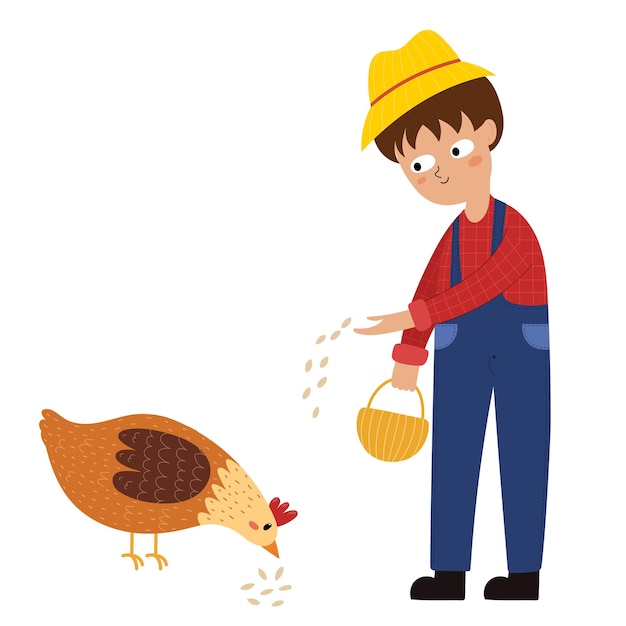This vibrant and colorful cartoon drawing depicts a young farmer boy feeding a chicken. The boy, with his brown hair and big eyes, is dressed in navy blue overalls that feature lighter blue pockets. He is wearing a red long-sleeve shirt beneath the overalls and black shoes. His outfit is topped off with a jaunty yellow hat that has a red rim. In his right hand, he holds a brownish-beige basket, and with his left hand, he scatters beige seeds onto the ground for the chicken.

The chicken, which is orange with a darker brown spot and tan feathers, is bending its neck to peck at the seeds. It has a red crest on its head, a yellow beak, and dark brown wings. The chicken stands on skinny beige legs as it enjoys the feed. The overall scene is one of pleasant agricultural activity, showing the boy's enjoyment of his task and highlighting the close relationship between the farmer and his livestock. The image is devoid of text, enhancing its universal appeal as a charming and lively depiction of rural life.